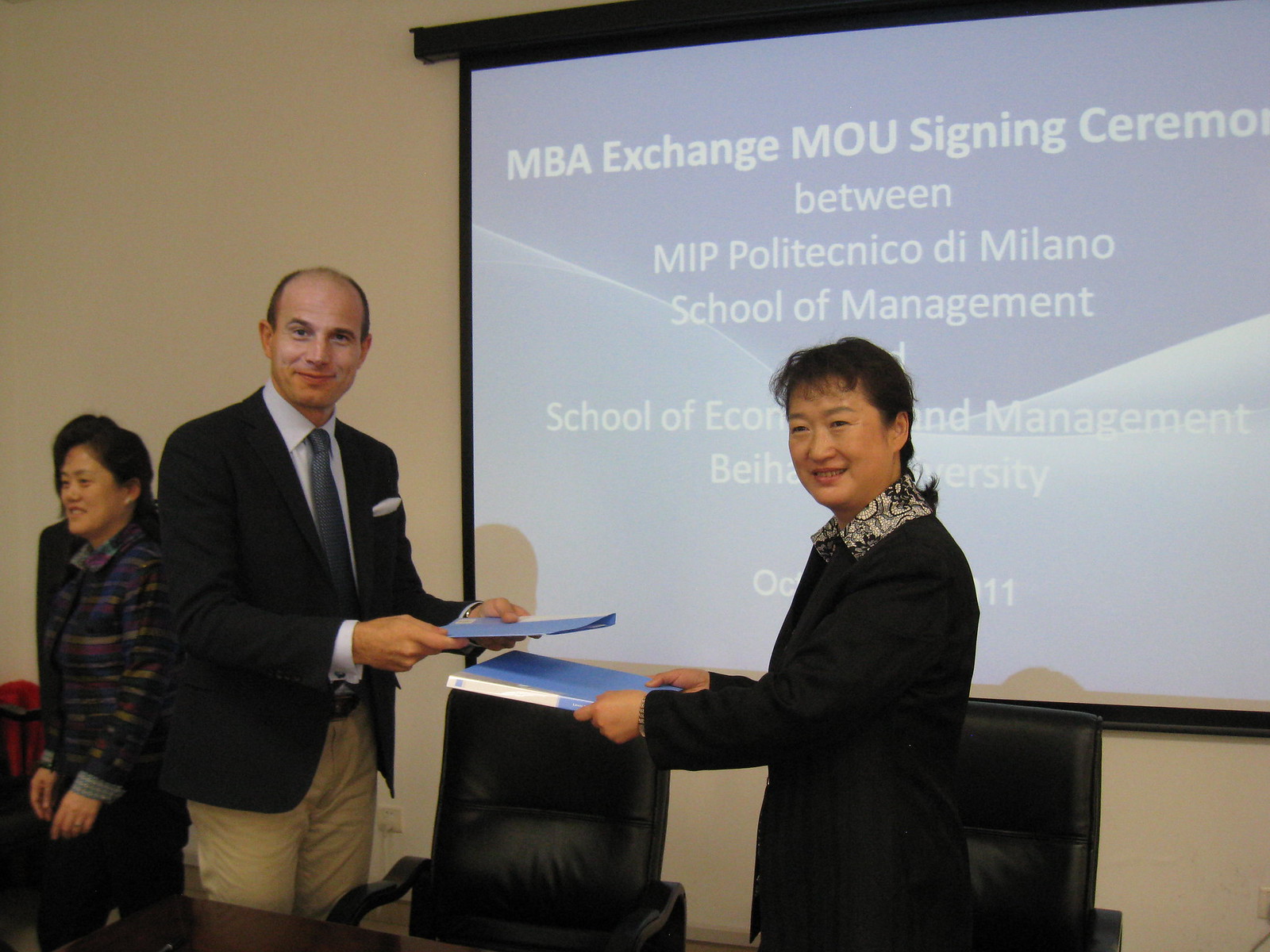The image captures a formal ceremony where three people are present. On the left side of the photo is a woman who is slightly out of focus and looking away from the camera, making her just barely visible. The main focus is on two people standing at the center, directly in front of a beige wall with a projector screen behind them. The screen displays a blue background with white text that reads, "MBA Exchange MOU Signing Ceremony between MIP Politecnico Di Milano School of Management and" but the remaining text is obscured by the individuals.

The man on the left is balding and appears to be in his 40s. He is dressed in khaki pants, a black jacket, and a gray tie. He holds a blue folder towards the woman on the right. The woman, who seems to be Asian and slightly older, is wearing a dark jacket with a decorative collar. She is also holding a blue folder, likely filled with papers, towards the man. Both individuals are smiling at the camera, symbolizing the formality and significance of the occasion.

In addition to these two primary figures, two black office chairs are visible in the background, adding context to the setting, which appears to be a conference room. The ceremony they are participating in is significant, likely involving an exchange of agreements between educational institutions, as indicated by the partially obscured text on the projector screen.